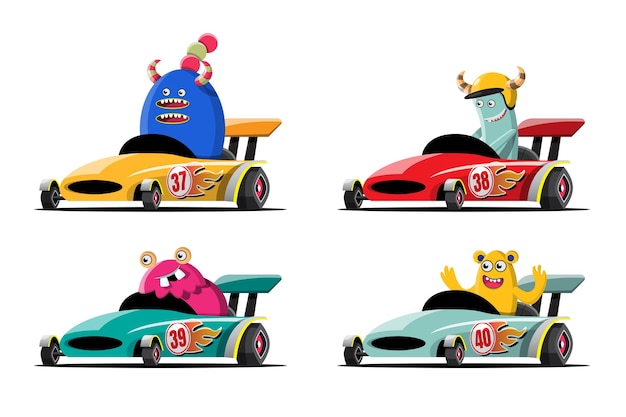This whimsical cartoon image features four small racing cars arranged in a 2x2 grid with no border or text, occupied by exuberant, unique creatures. In the upper left, a yellow race car marked with the number 37 and decorated with a flame is driven by a blue, oblong creature with two mouths, two eyes, and striped red and white horns. It also has three colorful spherical structures on its head. The upper right showcases a red car labeled 38, piloted by a cheerful green critter resembling Gumby, wearing a yellow helmet adorned with brown and white striped horns. The bottom left features a green car numbered 39 with a flame detail, ridden by a large, dark pink character with snail-like eyes on stalks and prominent buck teeth. Finally, the lower right displays a light green car marked 40, driven by a jubilant yellow character with its hands raised in the air and a broad smile. Each character exudes joy and excitement, adding to the playful and vibrant atmosphere of the scene.